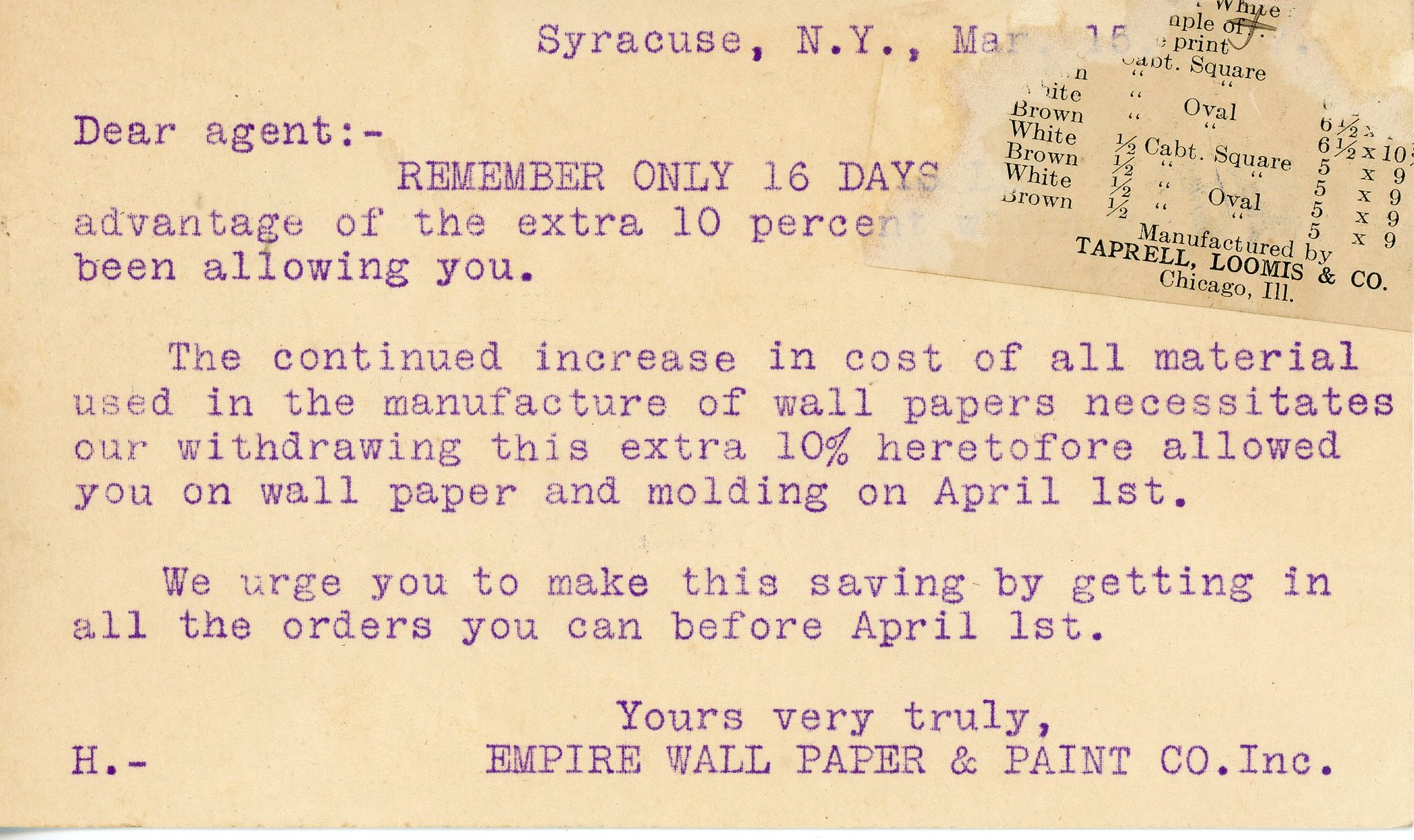The image is a rectangular telegram or letter, typed in a purplish-black ink on a yellowish, cream-colored paper. At the very top, it reads "Syracuse, NY, March 15th." The body of the text starts with "Dear Agent, remember only 16 days left to take advantage of the extra 10% we've been allowing you. The continued increase in the cost of all materials used in the manufacture of wallpaper necessitates our withdrawing this extra 10% heretofore allowed to you on wallpaper and molding on April 1st. We urge you to make the saving by getting in all the orders you can before April 1st. Yours very truly, Empire Wallpaper and Paint Co. Inc." The letter is signed off in the bottom-left corner with a capital "H" followed by a period and a dash. In the upper right-hand corner, partially covering the date, is a smaller piece of paper resembling a receipt or measurements, displaying dimensions and colors, labeled "Manufactured by Tarpell Loomis & Co., Chicago, Illinois." The image has a vintage, advertisement-like quality enhanced by the typewriter-style text and the textured background.